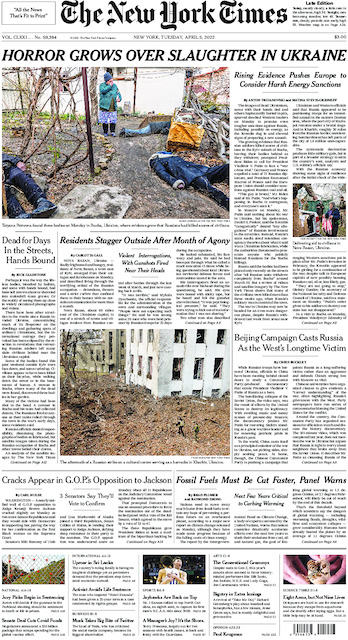The image depicts a New York Times article, distinguished by its recognizable logo at the top. The newspaper is unfolded, revealing a prominent, harrowing photograph of two bodies lying on the ground, an apparent scene of death. A person stands nearby, observing the bodies, and a third body is visible on the ground. The article's headline reads "Horror Grows Over Slaughter in Ukraine," with subheadings detailing the grim situation: "Dead for days in the streets, hands-bound" and "Residents stagger outside after month of agony."

The image is a stark portrayal of the war-torn region with photographs of a decimated apartment building, people navigating the dirt and debris outside, and the widespread devastation. Another article on the same page is titled "Boeing Campaign Casts Russia as the World's Long-time Victim," indicating a broader geopolitical perspective.

Towards the bottom of the newspaper are small, unrelated articles. One image shows a decorated fence, another depicts what seems to be an athlete, and the last one shows a hand holding an object. A UPC code is clearly visible in the lower right-hand corner of the newspaper, marking the issue for retail sale.